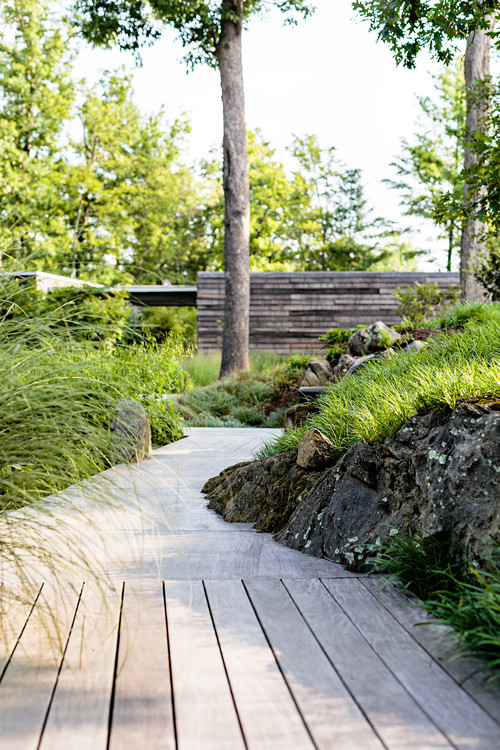The photograph, taken during the day in portrait orientation, captures an outdoor scene with a wooden walkway that leads through a natural setting. The walkway, made of gray wooden planks, starts at the foreground and meanders into the distance, eventually transitioning into a concrete path. Flanking the walkway are areas of dirt, grass, various plants, and rocks with patches of moss. Central to the image is a tall, prominent tree, with another large tree positioned more to the right. In the background, partially obscured by dense green shrubbery, a structure that appears to be a house peeks through. Beyond this structure, additional trees are visible against a backdrop of a clear, cloudless blue sky. A brick or possibly wooden wall with horizontal striations is also discernible in the upper third of the image, adding to the rustic, natural ambiance.